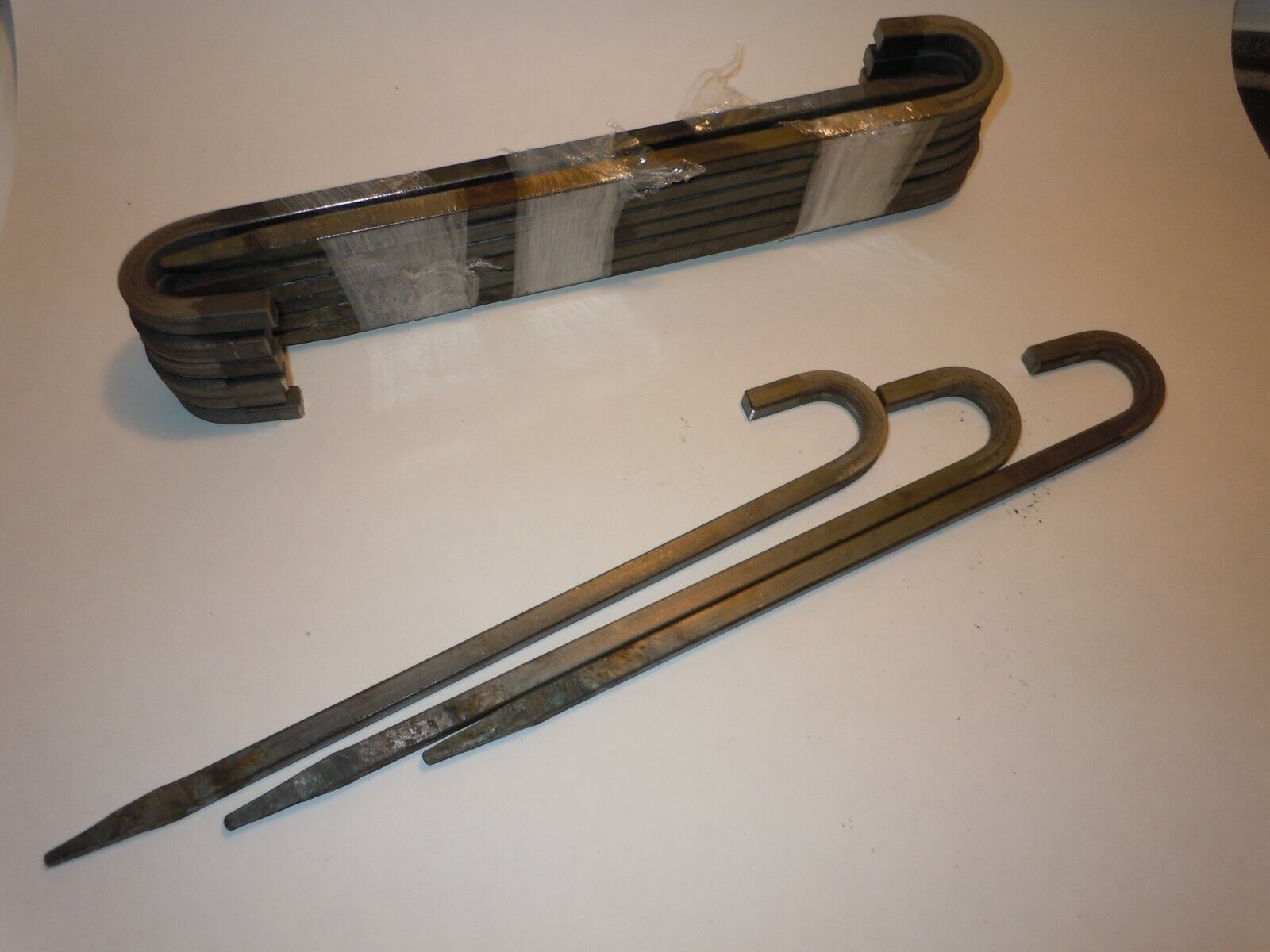In this photograph, we see a collection of metallic instruments placed on a light gray or tan-colored surface under low lighting. At the bottom of the image, there are three similar iron or steel hooks lying next to each other. These tools resemble elongated canes with one end being sharp and pointed, and the other end curving like a hook. Their surface exhibits shades of dark brown and gray. Higher up in the image, a larger bunch of these hooks is stacked vertically and secured together with clear plastic wrapping around their midsections. The contrast in arrangement and the distinct grouping provide a structured display of these utilitarian, road-like instruments.